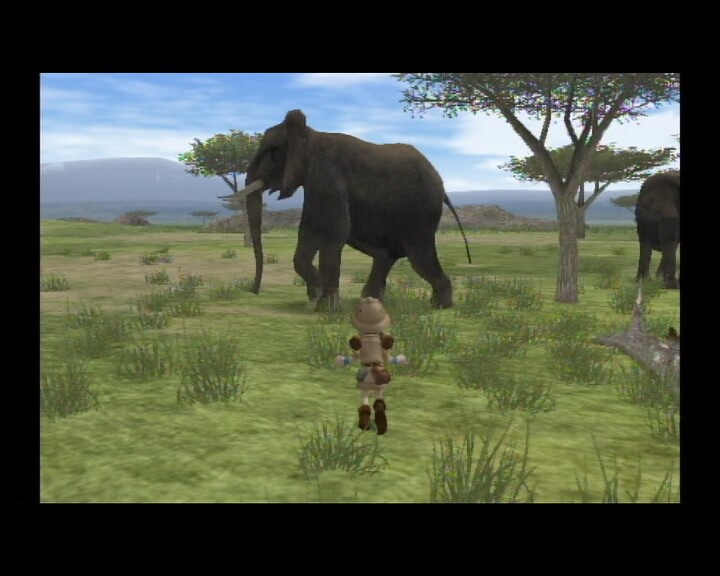In this landscape-oriented drawing, a small figure, seen from behind, dons a brown safari hat and matching attire, complemented by dark brown boots. Standing not far ahead is a towering mature elephant with impressive tusks, positioned between two trees—a large one on the right and a smaller one on the left. The backdrop features distant mountain ranges beneath a blue sky adorned with fluffy clouds, adding depth to the scene. The ground is a grassy terrain with sporadic tufts of weeds, capturing the rustic essence of the setting. To the right of the larger tree, a portion of another, slightly smaller elephant is visible, hinting at a serene coexistence amidst the natural landscape.